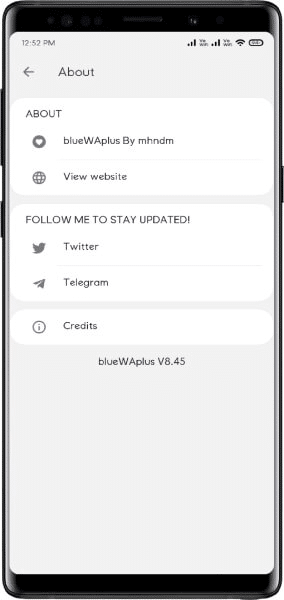The image features a smartphone displaying various app information and settings. In the upper left corner of the screen, the time is shown as 12:52 PM. On the upper right corner, icons for Wi-Fi signal strength and battery level are visible. The power button is located about a quarter of the way down on the right side of the phone, while the left side houses the volume up and down buttons.

Beneath the time, there is a left-pointing arrow accompanied by the word "About." Directly below this, a white rectangular section contains the header "About" in the upper left corner, along with a heart icon. This section also includes the text "Blue WA Plus by MHNDM." 

Underneath this rectangle, there is an icon resembling a globe, followed by the text "View Website." The screen then displays a second white rectangular section. At the top left of this section, it reads "Follow me to stay updated," alongside a Twitter bird icon and the word "Twitter." Adjacent to this is a paper airplane icon next to the word "Telegram."

Further down, there is a long, narrow rectangle featuring an eye icon within a circle, accompanied by the text "Credits." Below this, "Blue WA Plus V8.45" is stated. The rest of the screen is a blank gray space.